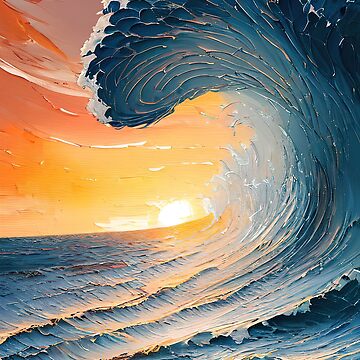This detailed oil painting captures the dramatic moment of an enormous, curling wave in the ocean during a sunset. The wave, depicted in a spectrum of blues ranging from light to dark, towers majestically as it forms a massive curl poised to crash. The crest of the wave is adorned with white foam, illustrating the forceful motion of the water. Beneath the wave and extending to the right, the ocean exhibits varying hues of blue, complete with textured ripples. The background showcases a vibrant sky where the colors transition from a bright white sun sitting on the horizon, extending into vivid yellow, and further blending into rich orange tones. Wispy white clouds add texture to the evening sky, contrasting with the warm sunset hues. This scene beautifully encapsulates the dynamic interplay between the powerful ocean wave and the serene, colorful sunset light, evoking a sense of warmth and summertime.